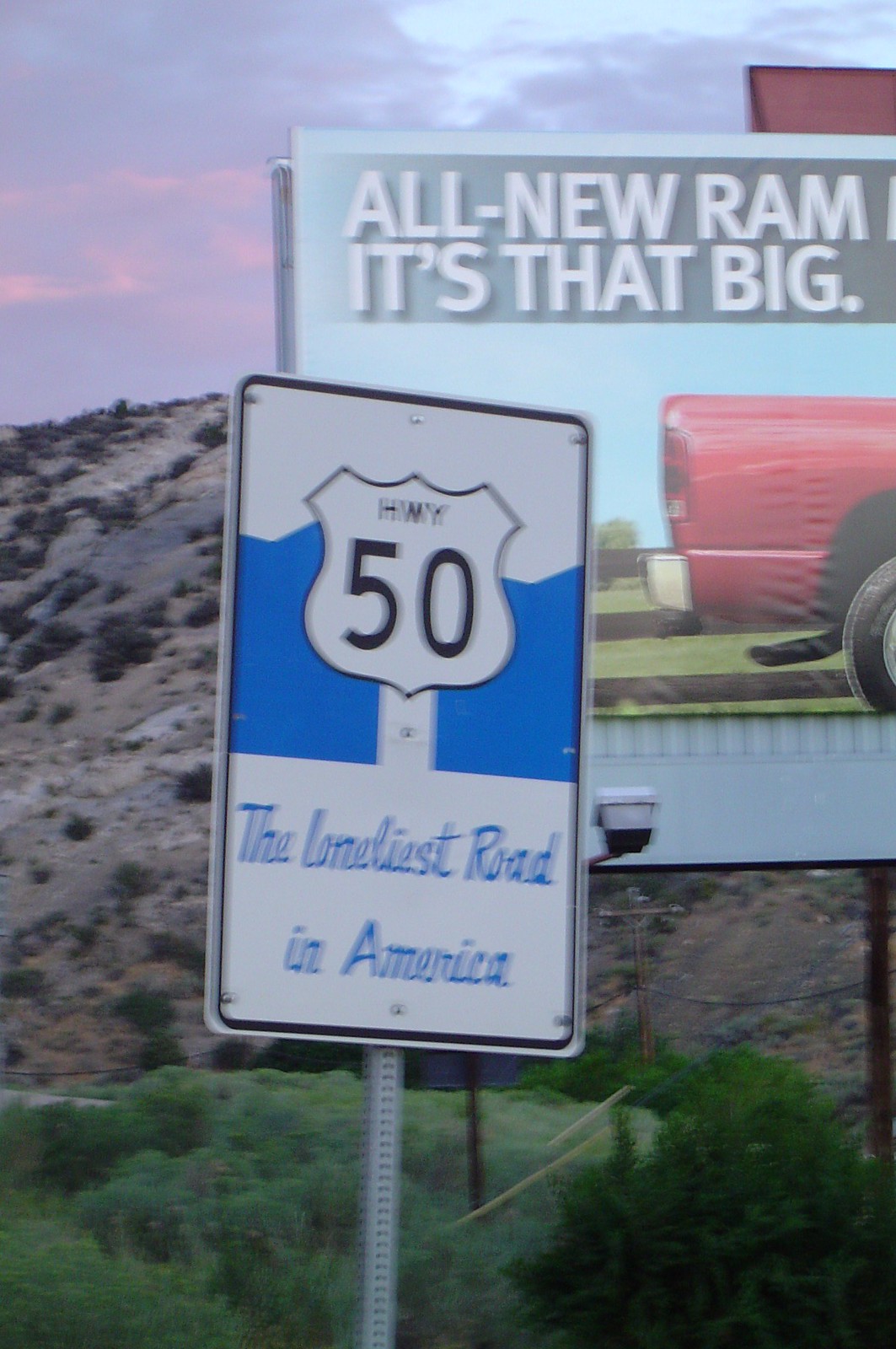This photograph, taken from a vehicle around sunset, captures a tranquil and somewhat desolate landscape. On the hillside in the background, there are patches of low shrubs and bushes, although the predominant colors are browns, tans, and grays, indicative of a dry terrain. The foreground is dotted with greener vegetation and rows of shrubs. A partially visible billboard occupies the left side of the image; it advertises the "All New Ram" and features a red truck, though only the rear portion of the vehicle is visible. Dominating the center of the photograph is a road sign mounted on a metal pole. The sign has a white background with black borders and prominently displays the U.S. Highway 50 shield. Beneath the shield, in blue letters, it declares "The Loneliest Road in America." Blue mountains provide a distant backdrop, enhancing the photograph's sense of vast, open space.